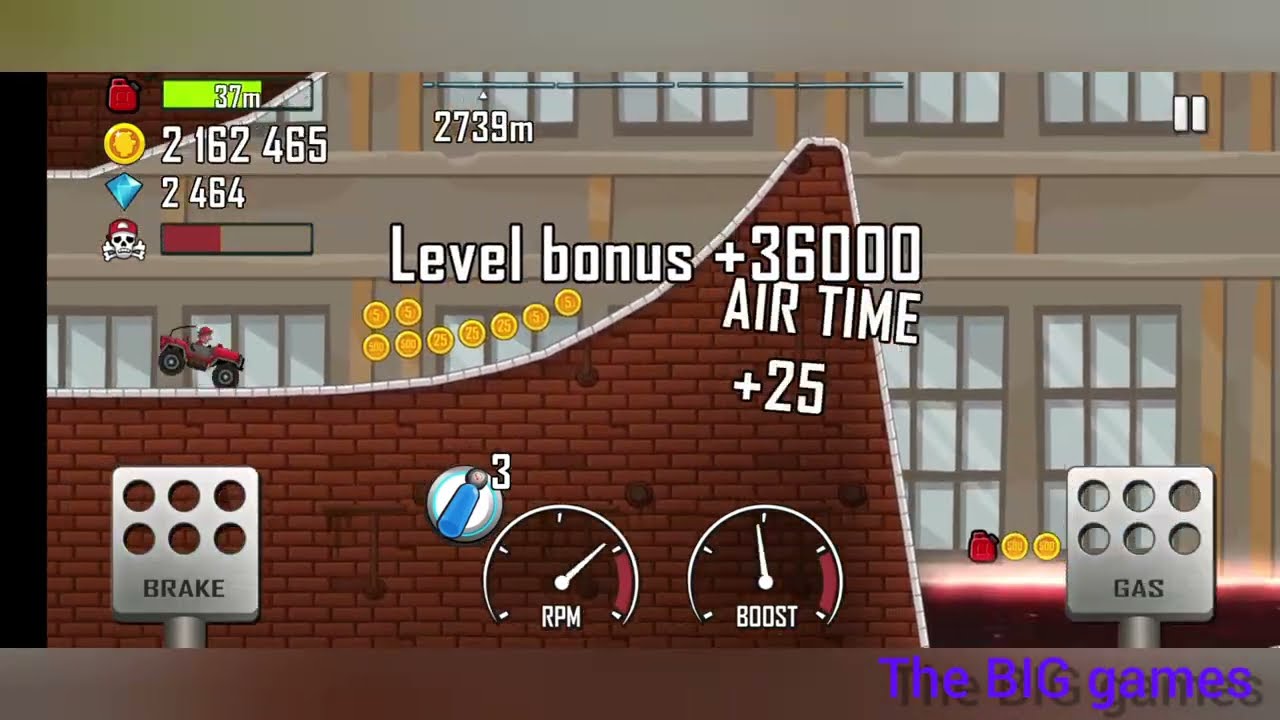This detailed screenshot appears to be from a mobile video game featuring a stunt-driving scenario. The central focus is a small red Jeep or a similar four-wheeler climbing a curved, dark burgundy brick wall, which has a white trim that slopes to a peak and then drops steeply. At the top center, a greenish-hinted gray line spans across, fading to a solid gray towards the right. The image prominently features various game elements, including two metal pedals on either side. The left pedal, marked "Brake," and the right, marked "Gas," each have three circular cutouts resembling a domino. Between the pedals are two gauges embedded in the wall, labeled "RPM" and "Boost." Above the Boost gauge are the texts "Level Bonus +36,000" and "Airtime +25," with a cluster of gold coins below. In the lower right-hand corner, there's blue text stating "The Big Games." The background showcases a gray building adorned with gold decorations and several tall windows. In front of the building on the right, a cylindrical metal structure with a sign reads "Gas." The setting encapsulates a dynamic and adventurous atmosphere, highlighting the stunt elements and in-game rewards.